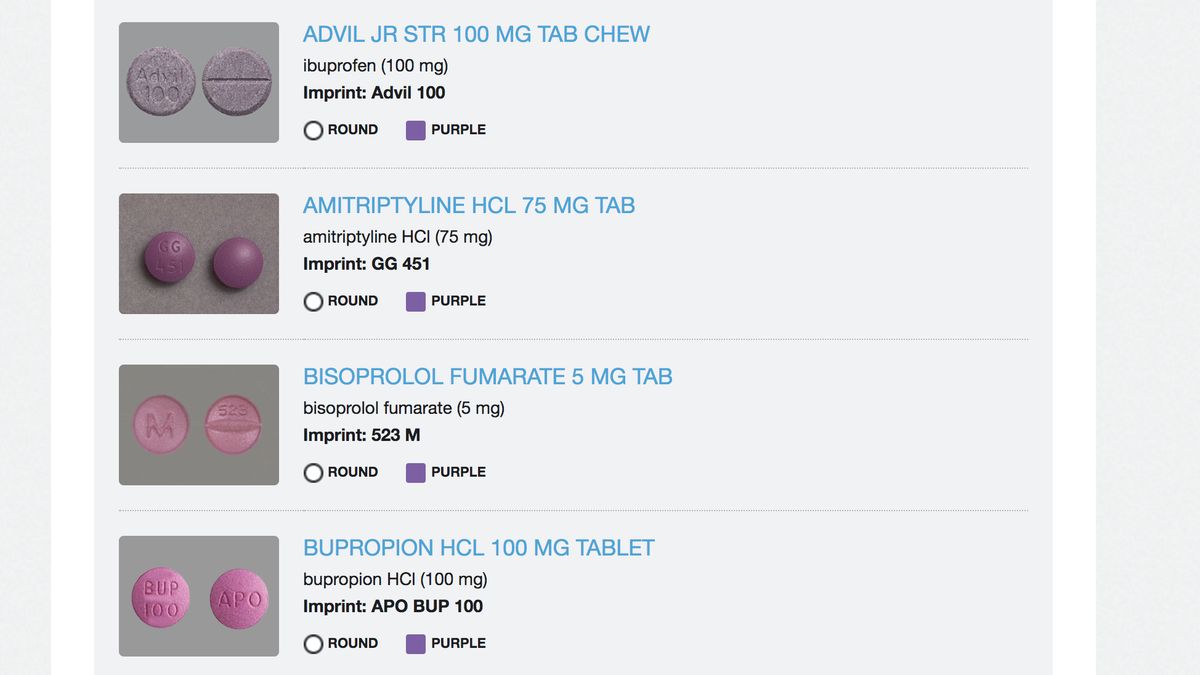This is a screenshot from a pharmaceutical search website. The website layout includes vertical gray rectangles on either side of the main content area, which features a light blue background. In the center, four search results for various medications are listed.

1. The first listing displays "Advil Jr. STR 100 mg Tab Chew" in blue font. To the left, there's an image of a chewable, grayish-colored pill. The text alongside the image states: "Ibuprofen 100 mg," and "Imprint: Advil 100," indicating that the pill is round and purple.

2. The second entry is for "Amitriptyline HCL 75 mg Tab." The accompanying text notes: "Amitriptyline HCL 75 mg," further specifying "Imprint: GG 451," indicating the pill is round and purple as well. There is a corresponding photo of this pill next to the description.

The detailed entries include the medication names, dosages, imprints, shapes, and colors, alongside images for easy identification.